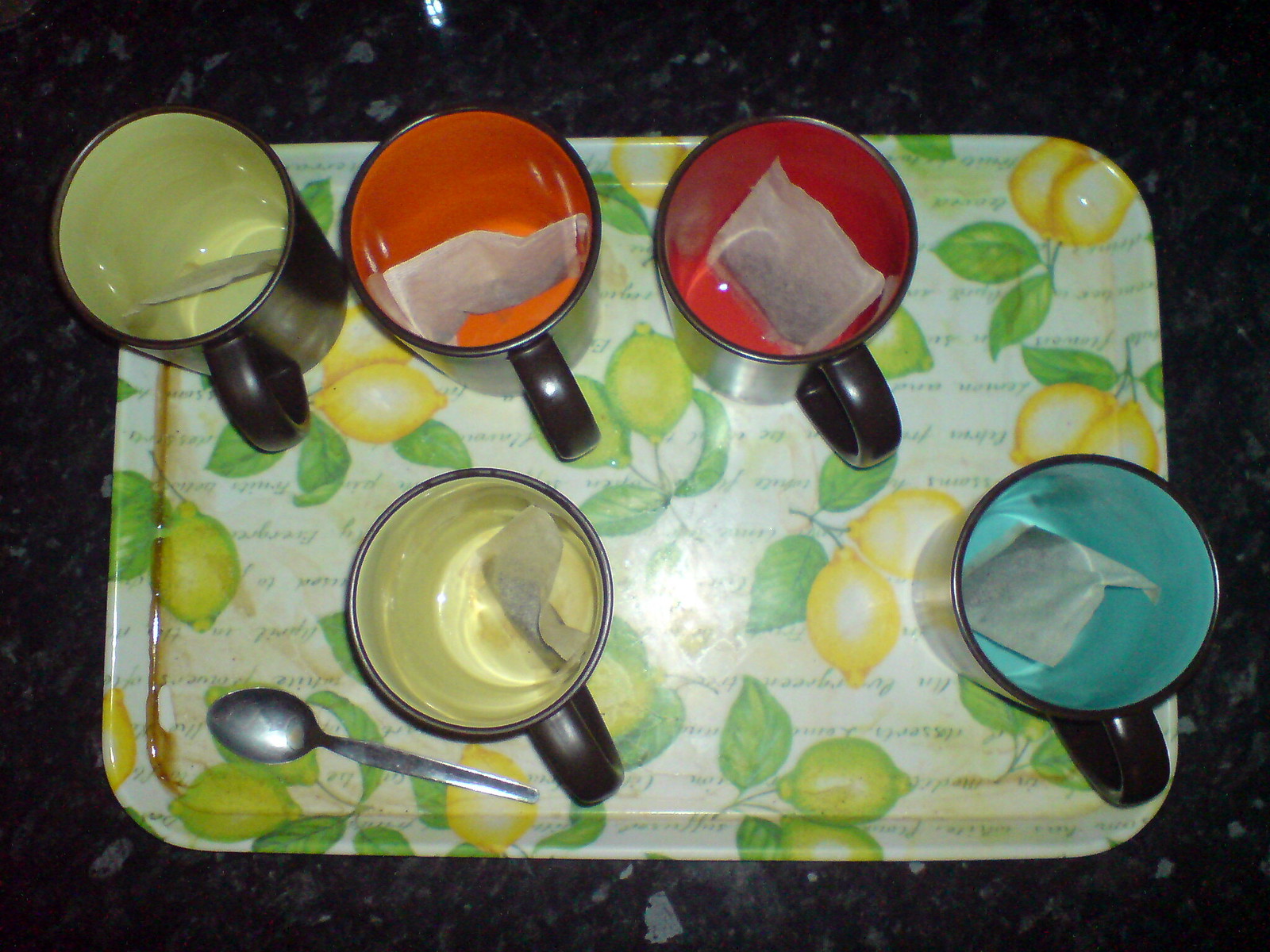This overhead photograph captures a vibrant tea setup on a serving tray decorated with lemon and lime illustrations and green leaves. There are five black ceramic drinking cups, each featuring a different-colored interior: two shades of yellow, one orange, one red, and one teal blue. Each cup contains a small tea bag and is arranged with three cups at the top and two at the bottom of the tray. The tray lies on a granite countertop, adding texture to the scene. Additionally, a silver spoon intended for stirring tea is placed in the bottom left corner of the image. The cups are empty, poised for hot water to be added, emphasizing the anticipation of a warm beverage moment.